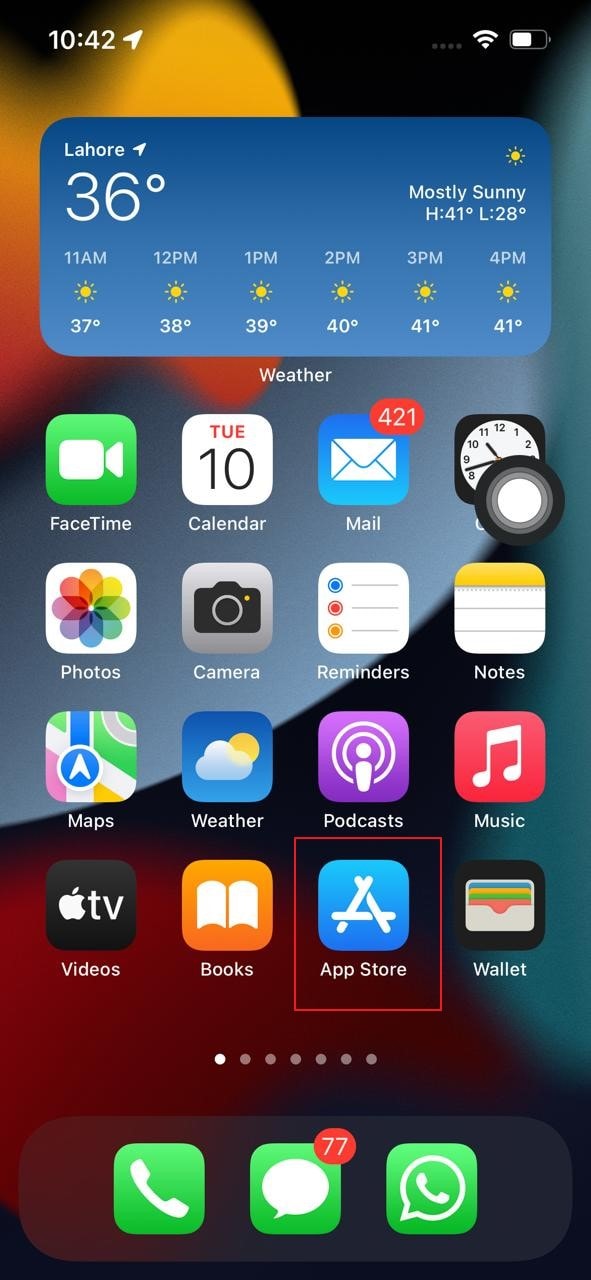The image captures an iPhone screen in meticulous detail. In the upper left corner, the time is displayed as 10:42. On the upper right, icons for the wireless connection and battery status are visible. Below this status bar, there's a weather widget showcasing the local weather in Lahore, indicating a temperature of 36 degrees Celsius. The widget also features a sun icon, suggesting it is mostly sunny with high and low temperatures forecasted at 41 and 28 degrees Celsius respectively.

The screen further displays an hourly weather forecast for the upcoming hours: 11 AM, 12 PM, 1 PM, 2 PM, 3 PM, and 4 PM. Each of these time slots is accompanied by a sun icon and an estimated temperature ranging from 37 to 41 degrees Celsius. 

Below the weather section, a series of app icons are clearly arranged. These include FaceTime, Calendar, Mail, Clock, Photos, Camera, Reminders, Notes, Maps, Weather, Podcasts, Music, Videos, and Books. Notably, the App Store icon is highlighted with a red border, followed by the Wallet app icon. 

At the bottom of the screen, there are three primary icons: a green box with a phone symbol, another green box with a speech bubble containing the number 77 in red indicating unread messages, and a third green box with a speech bubble enclosing a telephone icon.

The overall screen layout provides a comprehensive snapshot of the iPhone's functionality, including essential utilities, communication tools, and local weather updates.